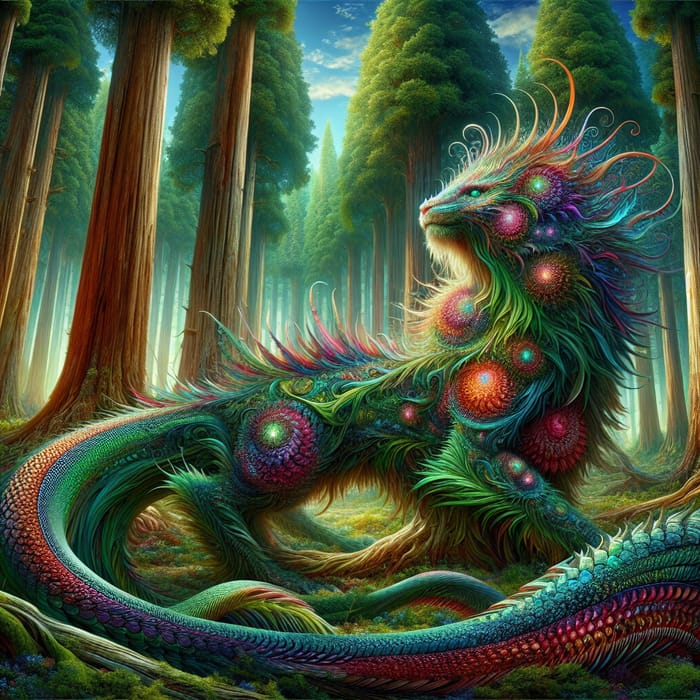In this digitally rendered, mystical painting reminiscent of a 90s Lisa Frank piece, a fantastical chimera meanders through a lush, dense forest adorned with towering sequoia and redwood-like trees. The deep blue sky, speckled with white clouds, bathes the scene in a dreamy, ethereal light. The mythic creature at the forefront boasts a vivid and complex array of features: the body and face of a cat with deep green fur and a serpent-like tail. Its fur shimmers with iridescent swirls of orange, green, blue, and purple, punctuated by glowing, flower-like orbs that resemble miniature galaxies. This creature, part dragon, part snake, exudes an abstract, otherworldly aura that is both captivating and surreal. The painting artfully blends elements of realism and fantasy, creating an enchanting visual narrative that draws viewers into its magical realm.